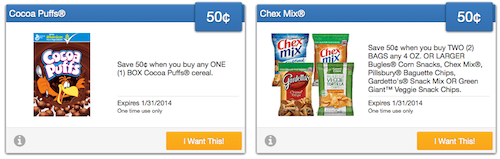The image is divided into two sections, each showing different promotional offers for cereal and snacks.

On the left side, there is a blue-outlined box featuring an offer for Cocoa Puffs cereal. At the top of this section, there is a small blue banner that reads "Cocoa Puffs," and a small blue box in the top right corner indicating "50 cents." The main portion of this side displays an image of a Cocoa Puffs cereal box, with the text stating, "Save 50 cents when you buy any one box of Cocoa Puffs cereal." The offer includes an expiration date which reads, "Expires on 01-31-2014." Additionally, within this section, there is a light blue box containing a gray circle with an 'i' icon on it located on the left, and a yellow button on the right that says, "I want that."

The right side of the image mirrors the left in layout but focuses on Chex Mix snacks. The top part of this section sports another blue banner, this time reading "Chex Mix," with a similar small blue box on the right indicating "50 cents." The main content here advertises, "Save 50 cents when you buy two bags of any 4 ounce or larger Chex Mix." In the lower left corner of this section, there is again a gray circle with an 'i' icon, and the right corner features another yellow button that says, "I want that."